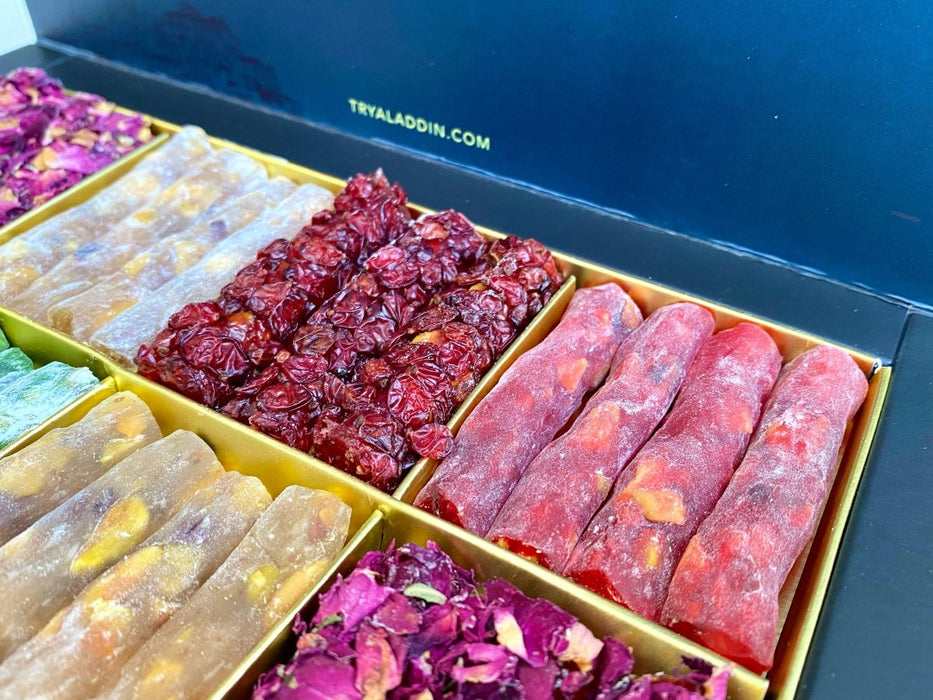The image is a color photograph, oriented in landscape, showcasing a bright blue box that contains six square trays lined with gold shiny foil, arranged at an angle from the top left to the bottom right. Each tray holds various rolled-up food items with diverse colors and textures. On the top right, there are reddish rolled-up dough items. Adjacent to these, moving left, the second tray contains what appears to be purplish leafy substances. To its left, a tray holds dark raisins, and further left, additional rolled-up white dough items. In the bottom row, the middle tray contains yellow rolled-up dough, while the bottom left tray holds light green rolled-up items. The bottom right tray features loose purple items. The background of the box's lid is dark blue with a prominent yellow text in all caps that reads 'TRYALADDIN.COM.' The image exudes a sense of photographic realism, capturing the vivid details and varied textures of the food items.